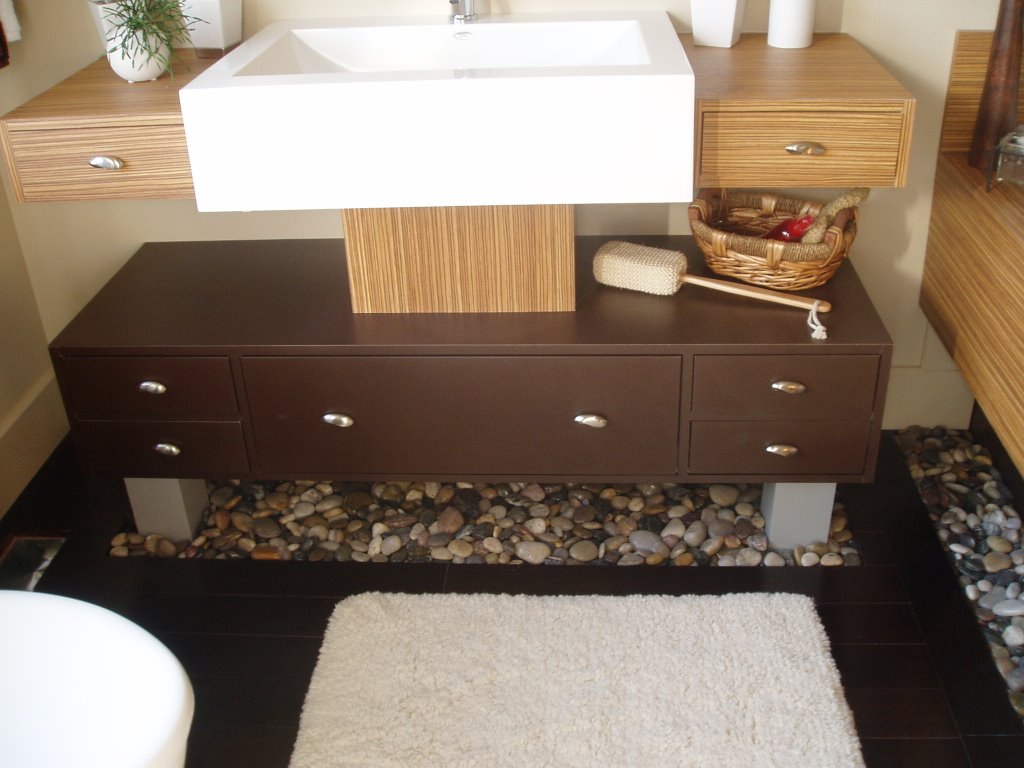The image showcases the interior of a modern bathroom. Central to the scene is a large white ceramic sink, elegantly mounted on a dark gray cabinet with a desk-like design. The cabinet features one long drawer in the middle and two small drawers on each side, all of which are supported by light gray legs. The flooring beneath is adorned with a vibrant pebble design, offering a textured look that could be either tiled or vinyl. Adding a touch of coziness, a white rug is placed on the floor.

To the left of the sink sits a vase filled with decorative twigs, adding an organic element to the contemporary decor. On the lower part of the cabinet, there is a sponge on a stick, equipped with a string loop for convenient wall hanging. Completing the bathroom setup, a basket filled with various soaps and shower gels rests on the cabinet. The arrangement presents an interesting mix of modern and natural textures that contribute to the room’s unique aesthetic.